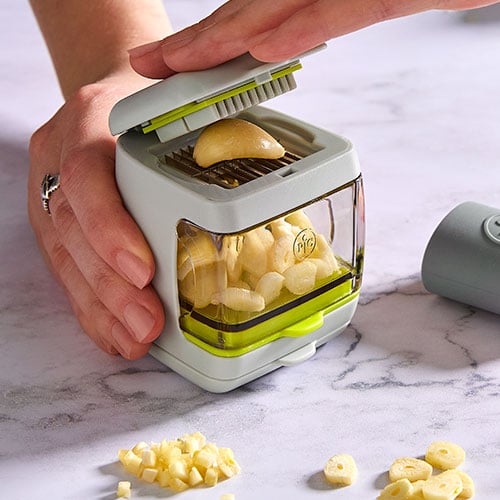A square box is depicted with a detailed white lid featuring ridges that flow downward and a green trim. The box itself has a transparent front, revealing a green tray at the bottom. Positioned prominently between the lid and the box is a whole garlic bulb, hinting at the device's functionality. This object appears to be a garlic slicer or crusher, designed such that pressing the lid crushes or slices the garlic, which then collects in the compartment below. The transparent area showcases a neat pile of garlic slices resting on the green tray. The scene captures a pair of hands actively engaged with the device — one holding down the box while the other exerts pressure on the lid. The entire setup rests on a pristine, white marble countertop adorned with additional chopped garlic pieces placed nearby, completing the context of a kitchen workspace.